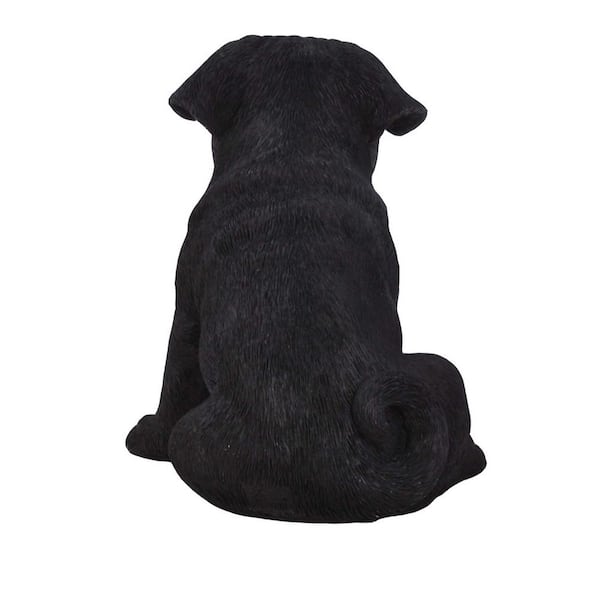The image features a small black dog, likely a puppy, sitting with its back towards the viewer on a pure white background. The dog has a shiny, smooth coat and appears to have big floppy ears that hang slightly over the edges of its head. Its short, curly tail loops almost into a complete circle and rests against its body. The puppy’s posture shows its left leg and paw extending outwards to the left as it leans slightly to the right, indicating most of its weight is on the left side. Wrinkles can be seen around its shoulders, hinting that it is still growing into its skin. The dog’s back is rounded, and its right haunch is slightly raised, with a glimpse of the right paw visible. Even though the scene is devoid of context due to the plain backdrop, the dog’s well-groomed, shiny fur and overall appearance give a lively and endearing impression.